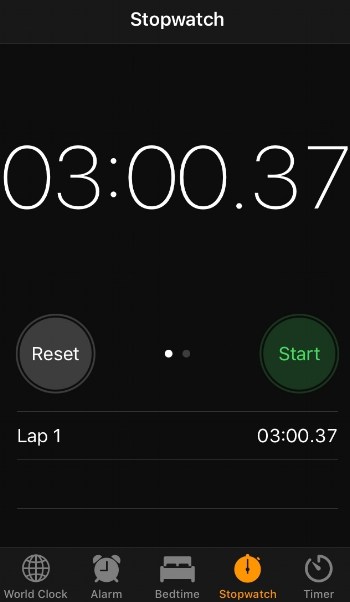The image displays a screenshot of the Clock app's Stopwatch section on a smartphone. The entire background is predominantly black, except for the bottom portion where the five app icons reside, which is dark gray. 

At the top center of the screen, the word "Stopwatch" is prominently displayed in white text. Below that, the stopwatch time is shown in a large font reading "03:00.37." 

Directly underneath the time, there are two buttons: a gray circle labeled "Reset" in white text on the left, and a green circle labeled "Start" in brighter green text on the right. Between these buttons are a small white dot and a gray dot indicating additional functions or statuses.

Further down, on the left side of the screen, the text "Lap 1" is labeled, and to the right of it, the same time "03:00.37" is displayed again. This section is separated by horizontal lines creating black rectangles.

At the very bottom of the screen are five app icons from left to right: World Clock (gray), Alarm (gray), Bedtime (gray), Stopwatch (highlighted in orange), and Timer (gray). These icons provide quick access to the different features of the Clock app.

The screenshot meticulously captures the user interface elements of the stopwatch feature, providing a detailed overview from top to bottom.